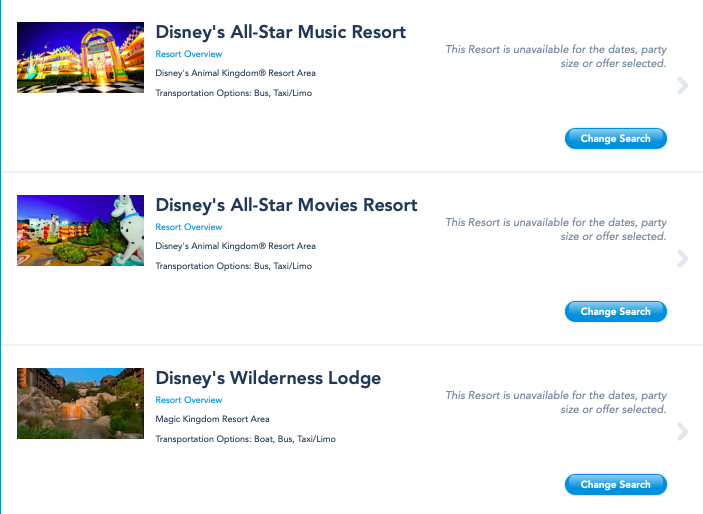This webpage from Disney showcases a list of Disney resorts, primarily distinguished by their thumbnails and brief descriptions. The page is designed with a clean white background featuring black type. 

At the top of the list is Disney's All-Star Music Resort, identified by a vibrant thumbnail photograph beside its name. Immediately below the resort name, written in blue type, is the label "Resort Overview." Further details include its location in the Disney's Animal Kingdom Resort Area and available transportation options such as Bus, Taxi, and Limo. To the right of the description, there's a notice indicating the resort is unavailable for the selected dates, party size, or offer. Next to this message, there's a gray arrow button for navigation and a blue "Change Search" button for altering the search criteria.

Beneath Disney's All-Star Music Resort is Disney's All-Star Movies Resort, similarly accompanied by a colorful thumbnail image. Below that entry is Disney's Wilderness Lodge, also represented with a thumbnail photograph. Each listing on the page carries an identical unavailability message, informing potential guests that the specific resort cannot accommodate their current search parameters.